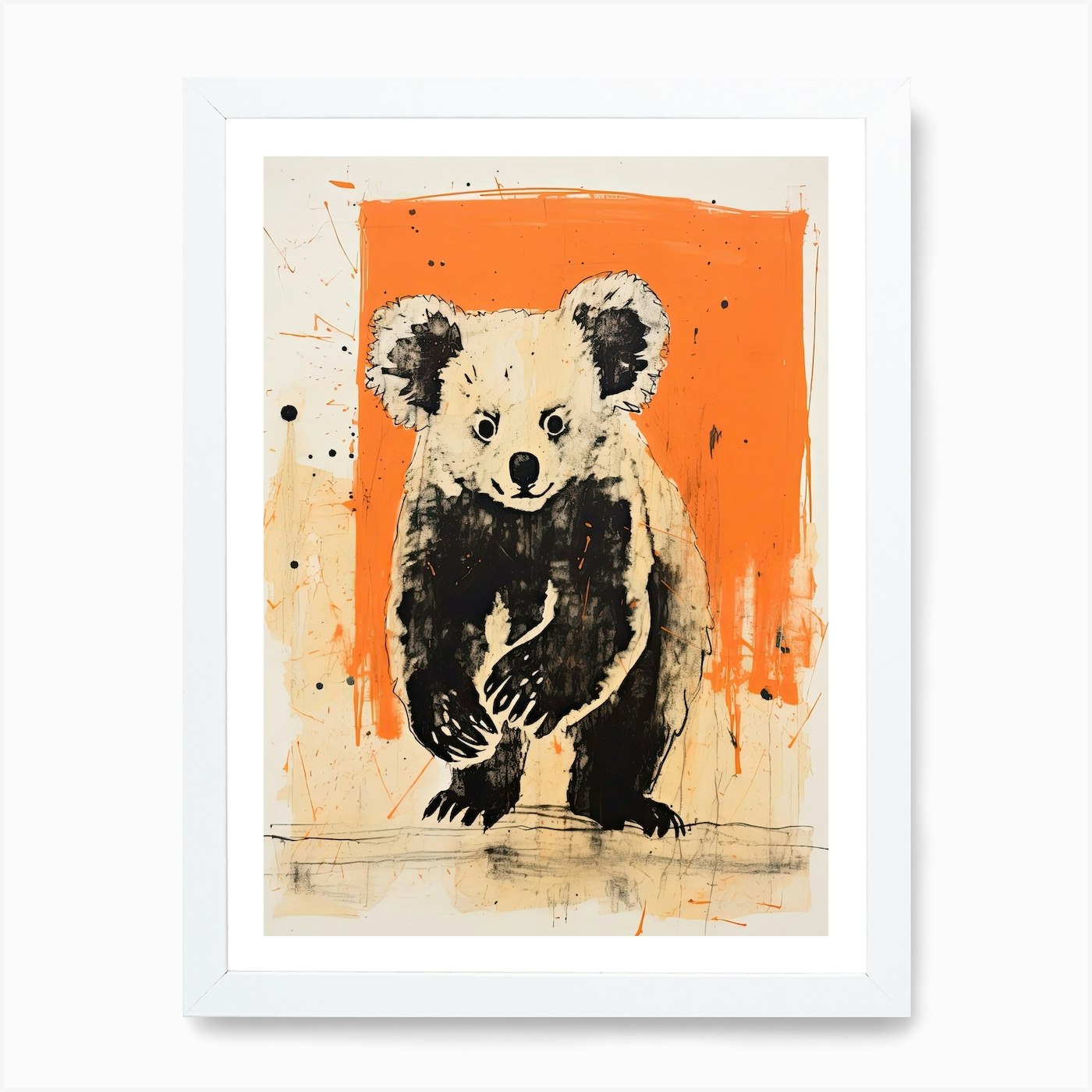The image is a painting of a bear cub, likely a panda bear, enclosed in a white frame with a white border and an off-white matting. The background features an orange rectangle, with some splotchy white-beige at the top and additional orange elements below. Ground beneath the bear is depicted with brown lines. The bear, rendered in an off-white and black palette, stands on its hind legs with its front paws off the ground. Detailed brushwork depicts its predominantly black fur with off-white accents, particularly on its face and chest. The bear's ears are dark, and it has striking black eyes, giving it a curious and intent expression as it looks directly at the viewer. The art style is splotchy, with vibrant strokes adding an impressionistic effect to the scene.